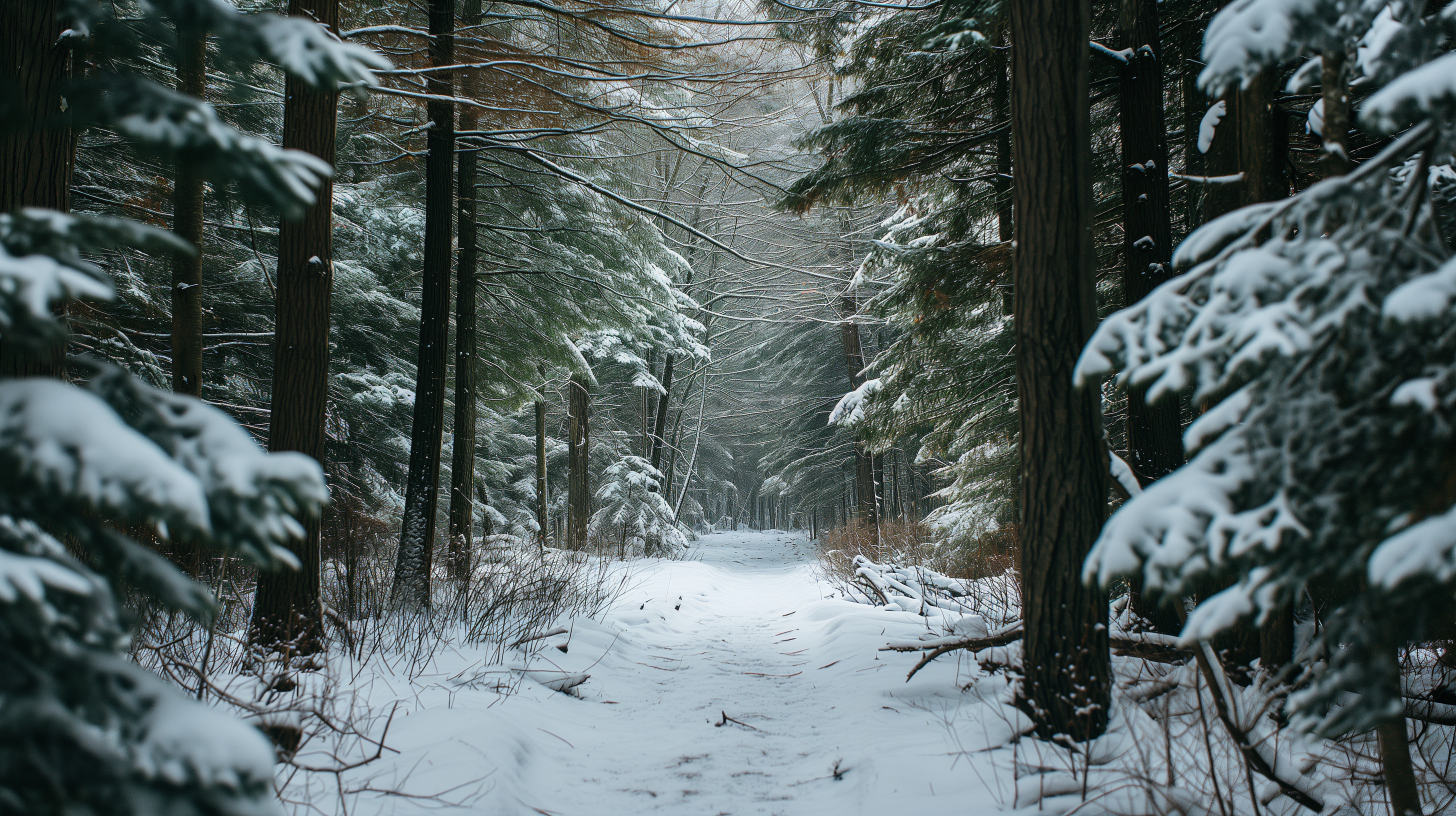The image depicts a serene winter forest scene taken at dawn, with a pathway that creates a tunnel-like effect framed by a diverse array of trees, including tall pines and oaks. The ground and branches are blanketed in freshly fallen white snow, with delicate flakes accentuating the green of the pine needles and the stark skeletons of dead twigs and sticks that litter the forest floor. Footprints of varying sizes meander down the snowy path, hinting at the presence of small animals, possibly visible in the distance with a dusting of frost on their brown fur. The path veers around a corner, inviting the viewer deeper into the woods, where the rich underbrush of red, orange, and brown twigs and grasses makes off-path travel challenging. The scene is tranquil and captivating, the blue dawn sky casting a gentle light over the pristine snowy landscape.